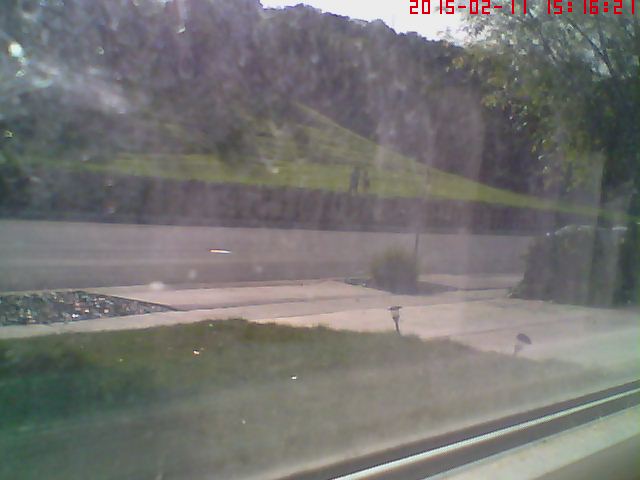This photo, taken from inside a home, offers an angled view of the front lawn. Dominating the foreground is a patch of tall, unkempt grass that spans the center and left portion of the image. The right side features a concrete driveway, receding into the background, bordered on its closer side by a rectangular band of gravel or small rocks. Alongside the driveway, there are two pathway lights: one leans over to the right while the other tilts slightly to the left. 

At the end of the driveway on the right side, a bush marks the boundary where it meets the sidewalk. The sidewalk horizontally intersects the driveway and extends to the left and right edges of the photo, leading the eye toward the background.

In the distance, a substantial green hill stretches across the image, enclosed by a lengthy fence that appears to be constructed of brick. Above the fence and to the right, the tops of dense trees are visible, adding depth to the scene. Lastly, in the upper right corner, a red digital timestamp reads "2015-02-11" and "15:16:21," marking the precise date and time the image was captured.